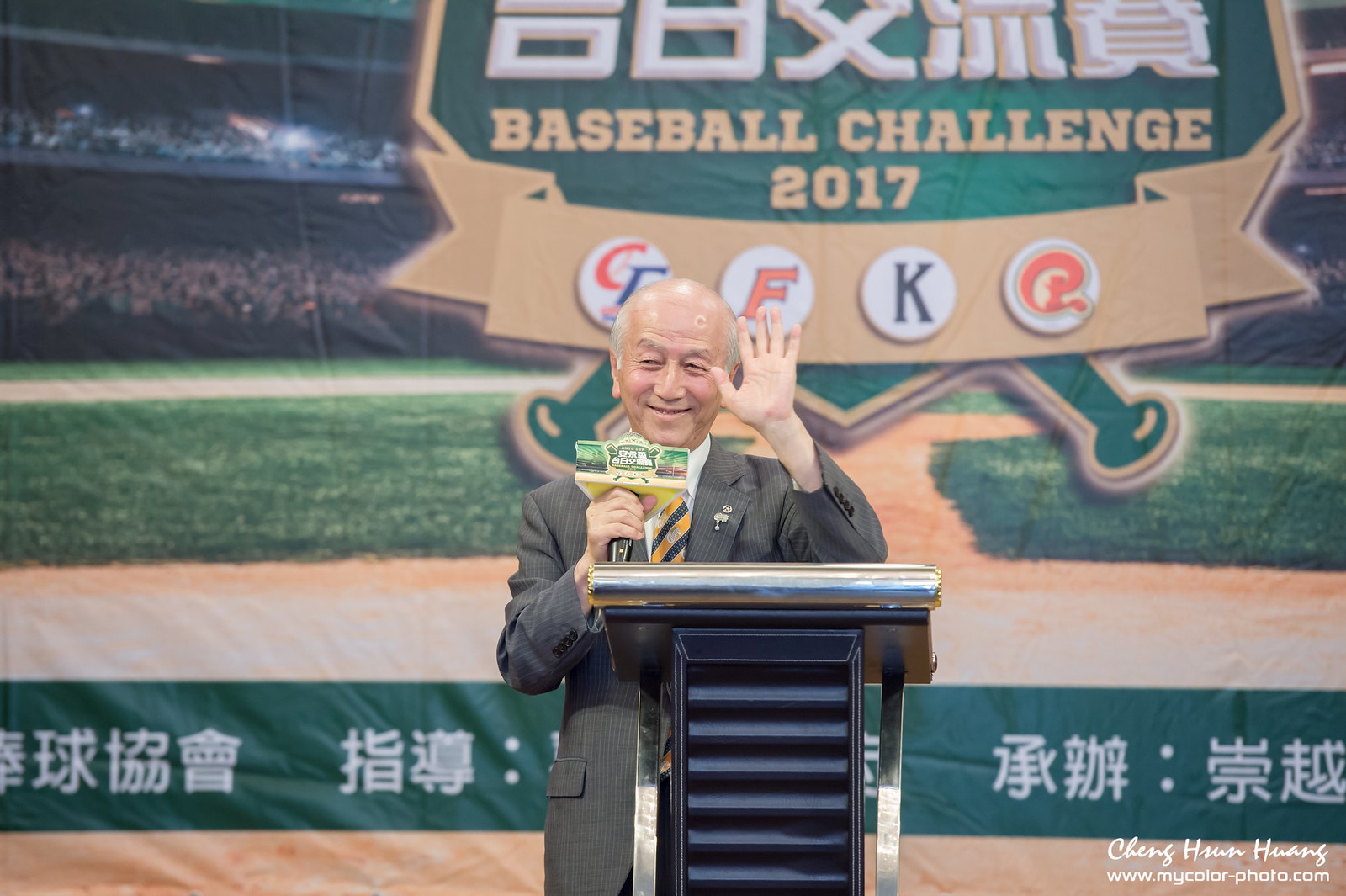The image depicts an older Asian man, likely in his 70s, standing at a blue podium with a green microphone that has a plastic attachment. He is smiling warmly and appears to be speaking, with one hand holding the microphone and the other possibly gesturing or waving. He has a graying, balding head with hair on the sides, and he's dressed in a gray pinstripe suit paired with a white collared shirt and a yellow-and-blue tie. Behind him is a large, vibrant banner showcasing a baseball field with visible bases, green grassy areas, and a stadium packed with blurry spectators in the stands. Prominently displayed at the top right corner of the backdrop is the text "Baseball Challenge 2017." The banner also features Asian characters and a tan ribbon with four team logos. At the bottom right of the image, the name "Chang Wong" and the website "MyColorPhoto.com" are noted.